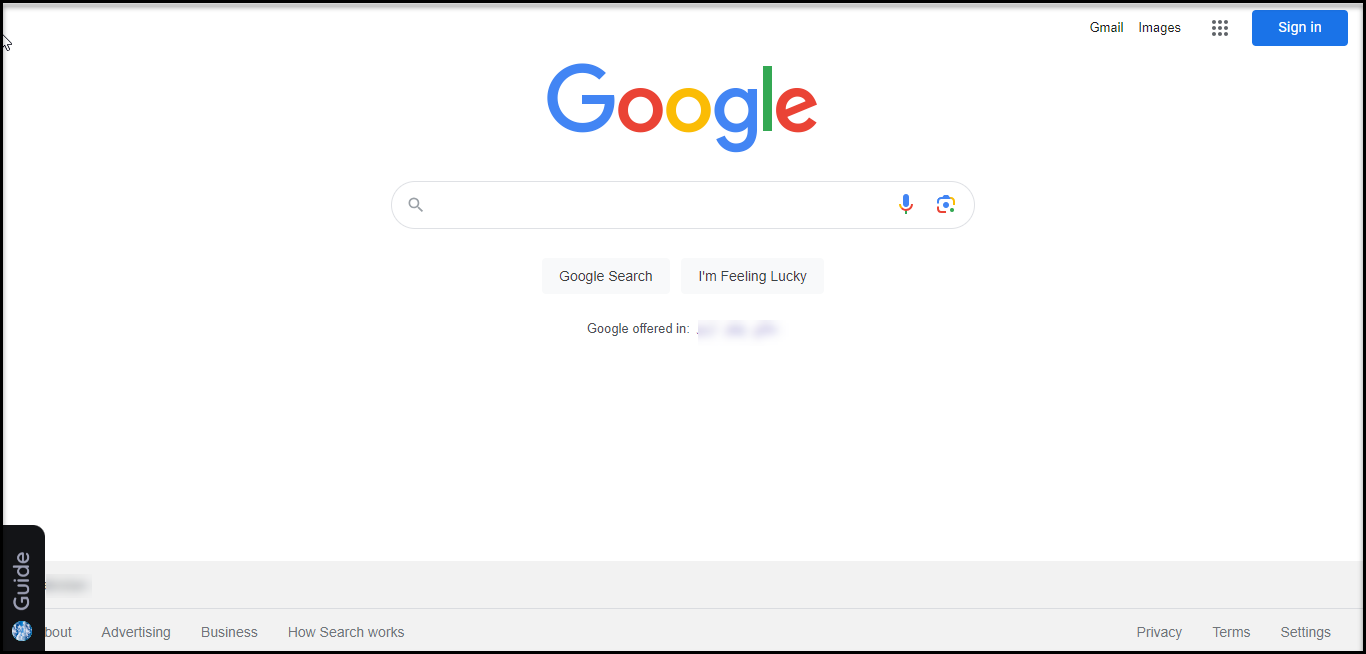This image showcases the classic Google homepage, characterized by its minimalist design. Dominating the center of the page, the iconic Google logo is prominently displayed above a single, expansive search bar. Below the search bar are two distinct buttons: "Google Search" and "I'm Feeling Lucky." Below these, the phrase "Google offered in" is visible with subsequent text blurred out.

At the top right corner, a navigation bar includes links to "Gmail," "Images," and a grid icon representing Google Apps. Also present are "Sign In" and "Sign Up" buttons. The layout is framed by a thin black border encompassing the main section.

In the bottom left corner, a black box labelled "Guide" is subtly visible. The footer of the page lists various links such as "Account," "Advertising," "Business," and "How Search Works," providing users with additional resources and information.